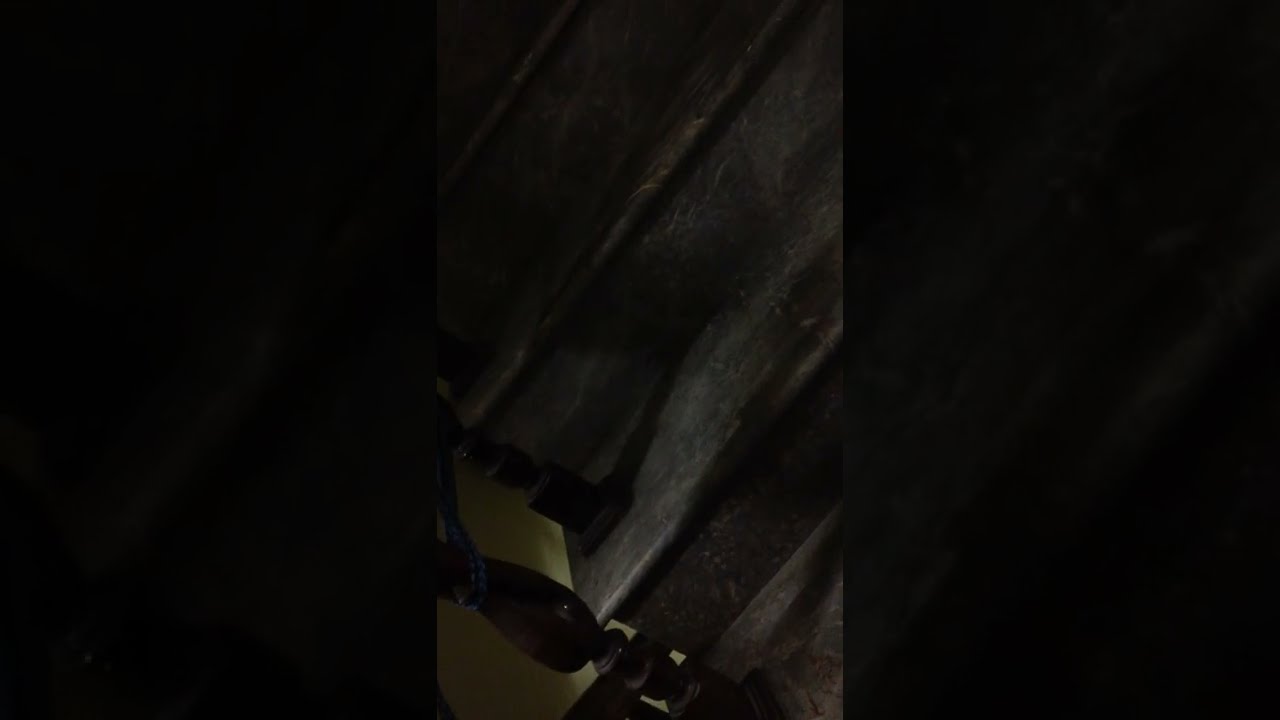This poorly-lit photograph, taken in portrait orientation and slightly tilted to the left, captures a close-up view of a stair made of black marble with edges that are curved. Dark brown wooden railings with a design pattern run alongside the stair, casting their shadows on the steps. Despite the darkness, hints of yellow in the image might indicate lighting or reflections. The edges of the image are bordered by two vertical black strips. The overall setting suggests an interior structure with elements resembling a wooden environment, possibly a basement with equipment, although the lack of clarity and additional context makes it challenging to discern definitive details.